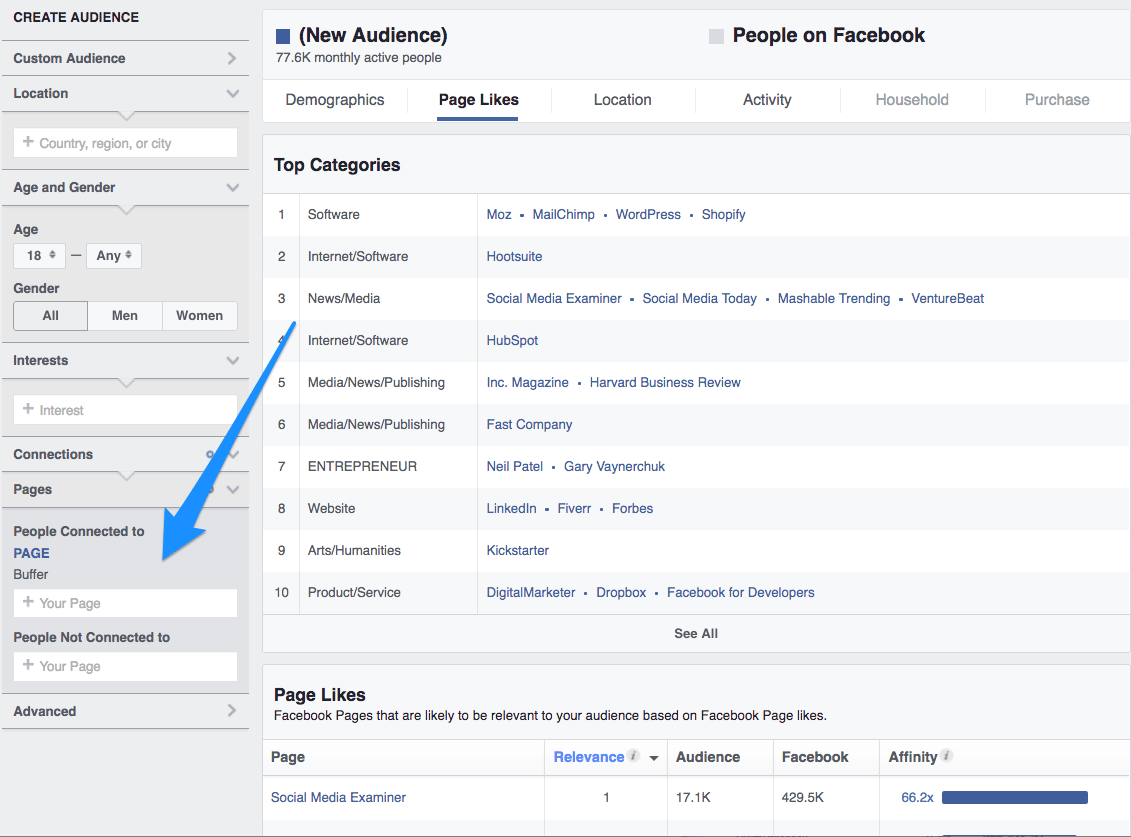In this image, a screenshot features a detailed interface against a white background dedicated to audience insights. On the left side, a gray vertical banner includes bold black text in the following hierarchy: "Create Audience" at the top, followed by "Custom Audience" with a right-facing arrow, and below it "Location" with a downward-facing arrow. 

Moving to the right, bold and large black text reads "New Audience: 77.6k Monthly Active People." To the right of this, there is a label "People on Facebook" followed by a horizontal menu of buttons placed against a white backdrop. These buttons, listed from left to right, are: "Demographics," "Page Likes" (which is underlined indicative of being the currently selected category), "Location," "Activity," "Household," and "Purchase."

Below this menu, a light gray banner displays "Top Categories" in bold text. Listed under this header are three main categories. Firstly, "Software" featuring associated entities such as Moz, MailChimp, WordPress, and Shopify. Secondly, "Internet Software" with Hootsuite noted to the right. Finally, the third category is "News Media" with an association to Social Media Examiner.